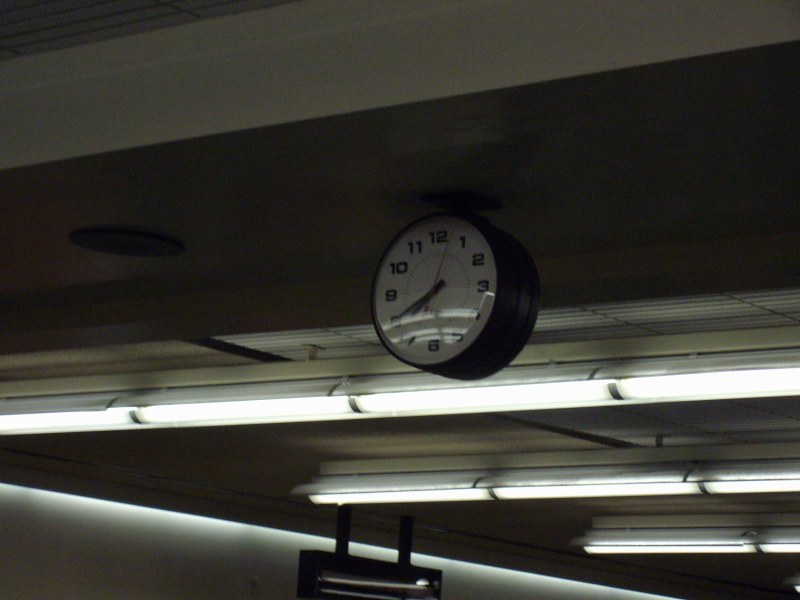A meticulously detailed photograph captures a ceiling-mounted clock, centrally positioned within a grid of metallic panels. The ceiling features horizontal white fluorescent tube lights that cast a bright, sterile glow across the image. Additional white lights are embedded beneath the edges of the wall, enhancing the overall illumination. The clock itself, hanging prominently from its top, showcases a classic design with a stark black border framing its white face. Bold black numerals encircle the clock, while the black hour hand and minute hand point to 8 and just before 8, respectively. The smaller red second hand is captured in motion, positioned just past the 12, conveying a precise moment in time.